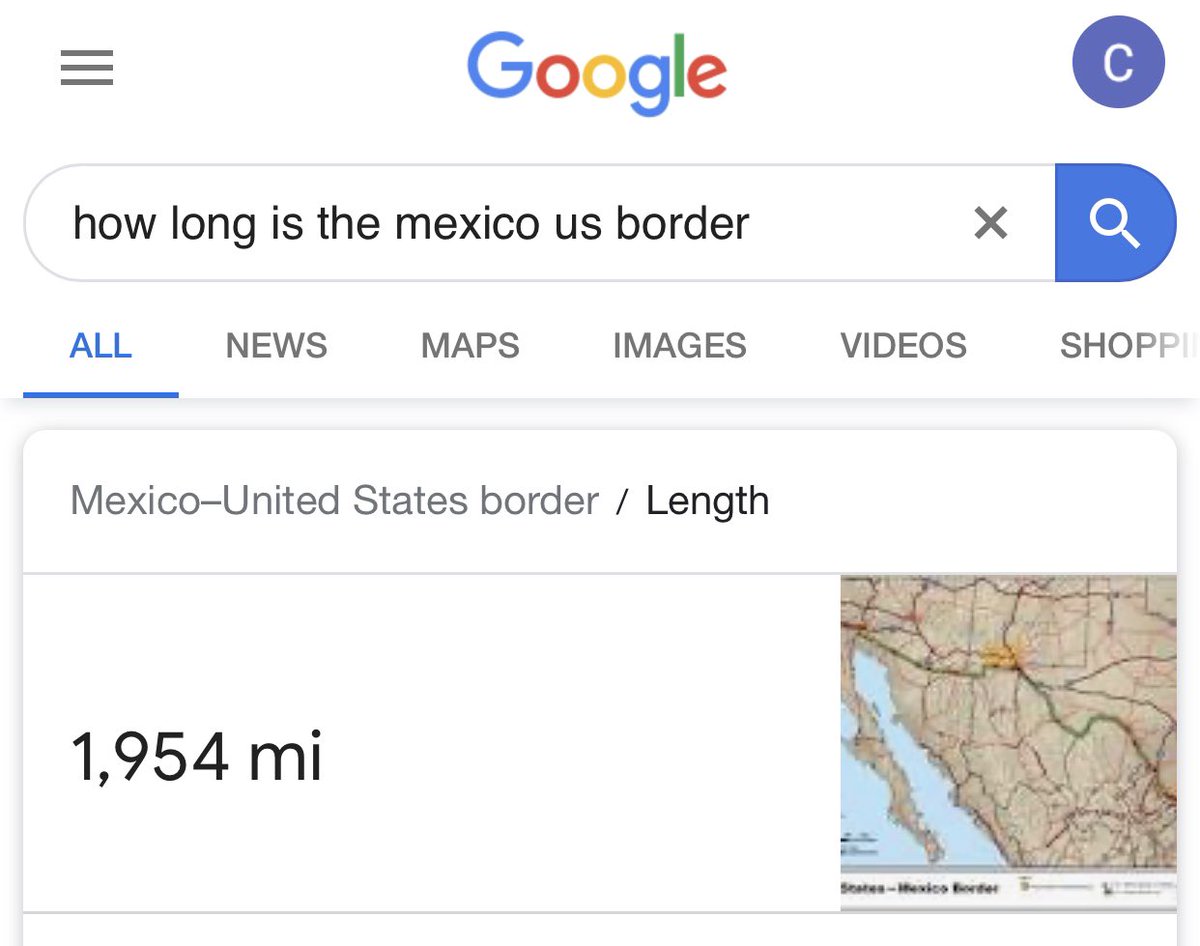This detailed caption is cleaned up and descriptive:

---

The image is a landscape-oriented screenshot of a Google search results page, predominantly featuring a white background. In the upper left-hand corner, there are three horizontal gray lines representing the menu icon. Centrally at the top is Google's main colorful logo. On the upper right-hand corner, there is a blue circle with the white letter "C" inside, indicating that a user is signed in.

Below this top row is the search bar where the query "How long is the Mexico-US border?" is typed. To the right of the search bar, there is a blue search icon, along with an option to exit the search.

Underneath the search bar, a horizontal navigation menu displays various tabs such as "All" (highlighted in blue and underlined), "News," "Maps," "Images," "Videos," and "Shopping," which are in gray.

The next section contains a large rectangular box with rounded corners. The top line within this rectangle states "Mexico-United States border / length." Directly below this, it states "1,954 miles" in bold text. To the right of this textual information, there is an image representing the Mexico-United States border, illustrating the border crossings and the extensive length of the border.